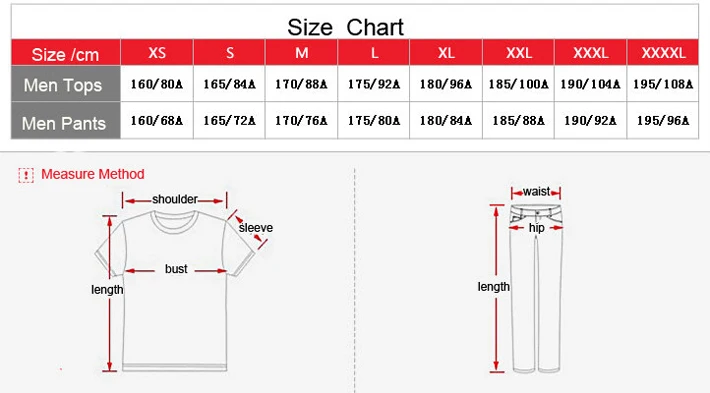This image is a detailed size chart for men's clothing, specifically tops and pants, displayed prominently on a website for online shopping. The top third of the image features a comprehensive sizing chart, with sizes ranging from XS to XXXXL listed horizontally. Directly below this are two separate sections: one for men's tops and another for men's pants, each detailing the specific measurements corresponding to each size.

The bottom two-thirds of the image focus on visual illustrations of a shirt on the left and a pair of pants on the right, each annotated with red arrows pointing to key measurement areas. For the shirt, arrows indicate the length (top to bottom), bust (left to right across the chest), shoulders (across the top), and sleeve length (down the right sleeve). The pants illustration similarly features arrows denoting the length (top to bottom along the left), waist (topmost horizontal measurement), and hips (horizontal measurement below the waist).

Additional text in the image includes "Measure Method" in red letters next to both the shirt and pants illustrations, emphasizing the importance of accurate measurements. The clear and concise layout, with black text for measurement labels and red arrows highlighting measurement lines, ensures that viewers can easily understand how to match their body dimensions with the appropriate clothing sizes.